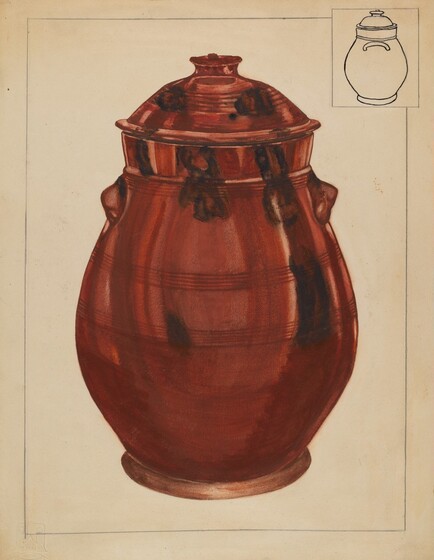This detailed drawing depicts an ancient urn or water pot, showcased on a cream or tan-colored background. Its reddish-copper hue implies it could be made of aged copper, evident from the subtle discoloration. The urn features a prominent, broad body that tapers towards the top, leading to a secured lid. Handles are positioned on either side just below the lid, though one handle is visible in a small, square inset in the top right corner. The urn's design includes some indistinct black and brown markings that may be decorative or a result of paint or aging. The entire illustration is framed by a thin pencil line, suggesting it comes from a detailed hand-drawn or pen and ink sketch possibly within a book. The base of the urn, matching its reddish-copper color theme, culminates in a goldish ring.